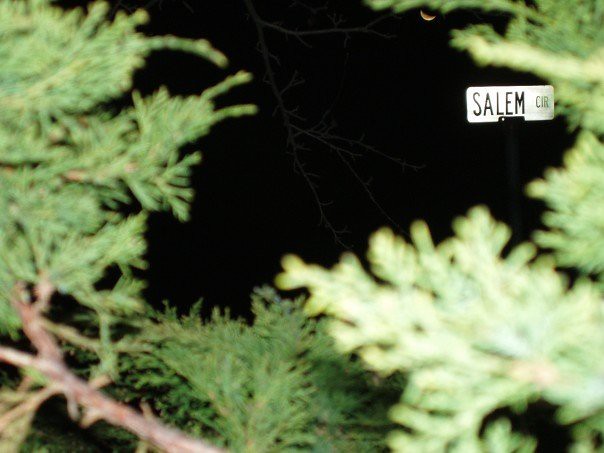This night image, captured through a dense cluster of bright green, out-of-focus pine branches with jagged edges, highlights a small section of a dark, unobstructed sky. Dominating the night sky is a thin, long tree branch extending out from the center, accompanied by a few smaller offshoots, casting an eerie silhouette against the blackness. Slightly to the right of the image's center, an orange-tinged crescent moon glows faintly, possibly altered in color by the lighting conditions. Near the upper right corner, a street sign marked "Salem Cir" stands out against the night, its white reflective surface illuminated by the camera's flash, mounted on a black pole. The natural frame created by the pine branches in the foreground adds depth and context, drawing attention to the sparse but striking elements beyond.